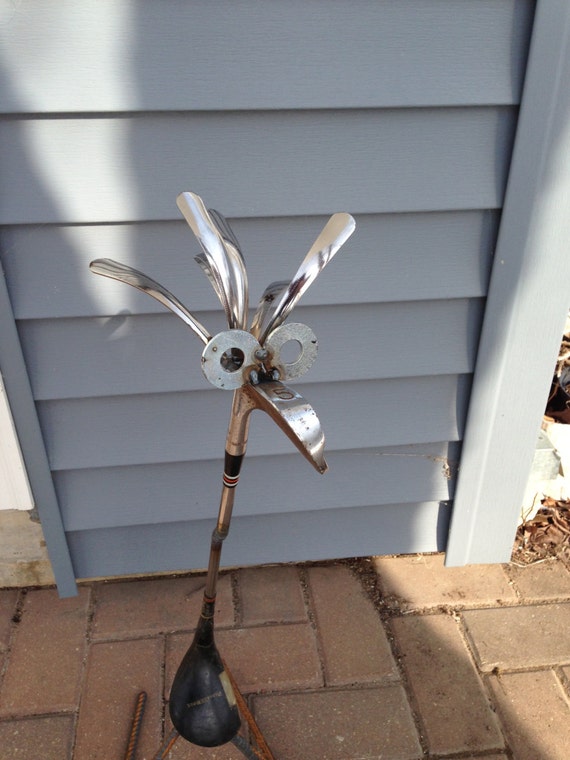This photograph captures an outdoor scene featuring a modern, stylized bird sculpture crafted from repurposed metal objects. The sculpture is situated on a brick paver surface, with sunlight casting shadows against a backdrop of a gray door and wall. The bird-like structure stands vertically, anchored by rebar twisted into the shape of legs. The base of the sculpture reveals a dark wooden golf club head. The main body consists of two welded golf clubs, where the top half is a putter with an attached handle, detailed with black, white, and red elements. Two metal O-shaped washers form the eyes, and various metallic utensils create a crest, giving the entire piece a whimsical yet artistic appearance.